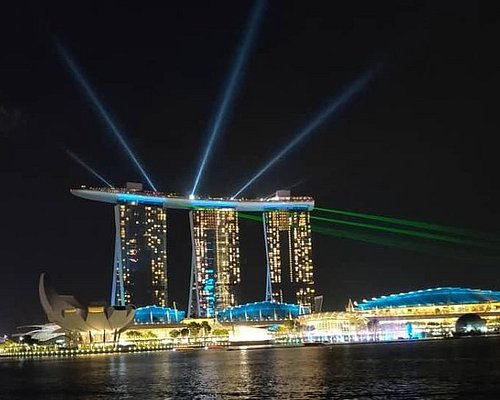This striking nighttime photograph captures a futuristic city skyline from the perspective of someone on a boat in a large body of water. The foreground features the calm water, leading to a brightly illuminated shoreline. Prominently, three high-rise buildings are connected by a spectacular rooftop structure that stretches across them, resembling a giant float. Each end of this rooftop emits brilliant white light, while a distinct green light extends from the right side of the structure. The city, renowned for its stunning architecture, is widely believed to be Singapore, showcasing one of its most famous landmarks.